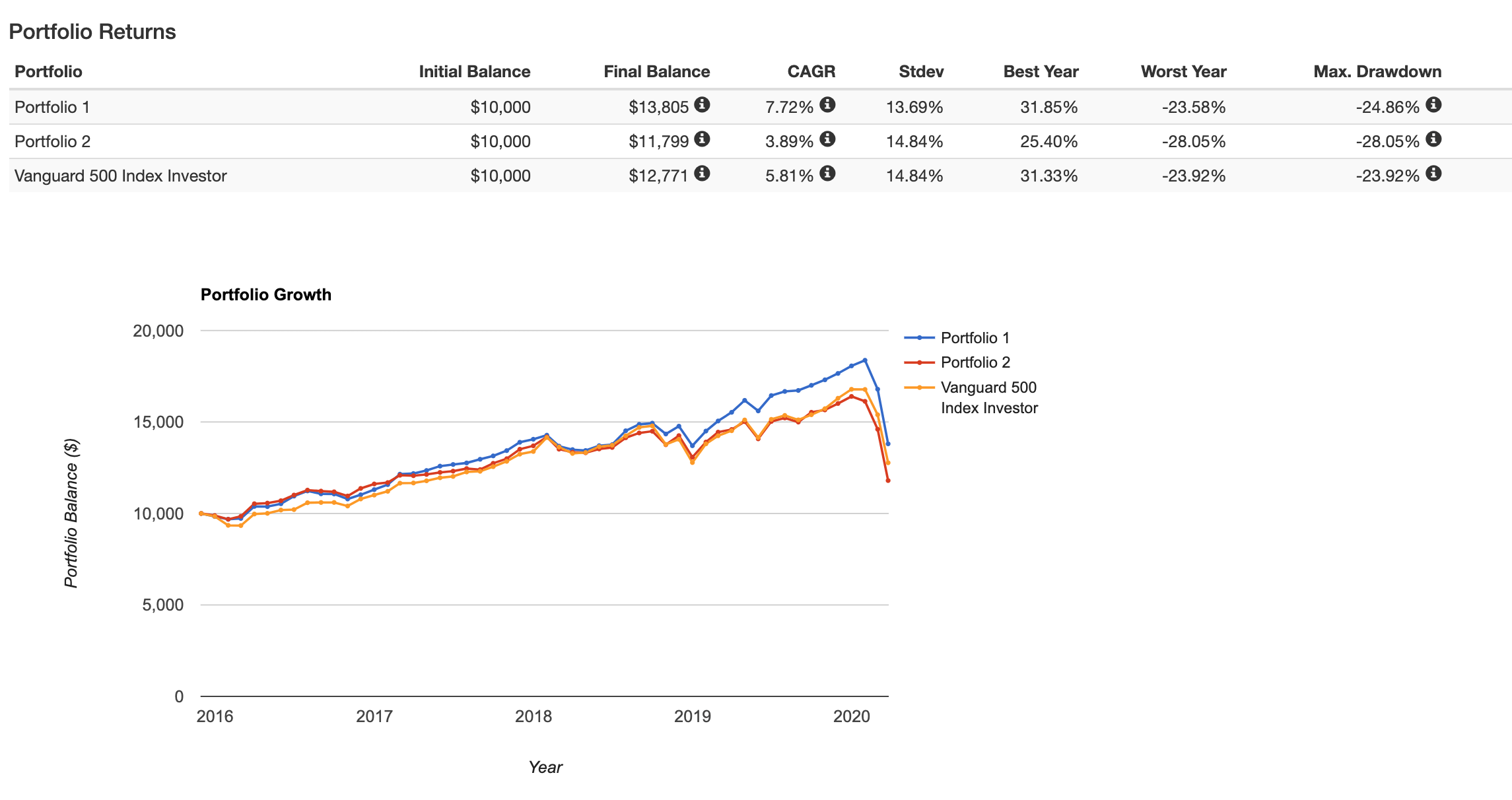The color image features a detailed comparison of three portfolios' investment performances. At the top, against a white background, is a table with black text detailing the portfolios' metrics. The table columns are labeled: Portfolio, Initial Balance, Final Balance, CAGR (Compound Annual Growth Rate), STDEV (Standard Deviation), Best Year, Worst Year, and Max Drawdown. The three portfolios listed are Portfolio 1, Portfolio 2, and the Vanguard 500 Index Investor, each with an initial balance of $10,000. Their final balances are $13,805, $11,799, and $12,771 respectively, with additional numerical data for the other metrics.

Below the table, there is a line chart depicting the performance of these portfolios over time. The x-axis ranges from the years 2016 to 2020, while the y-axis marks the portfolio balance in dollars, ranging from $0 to $20,000 in $5,000 increments. The chart's lines are color-coded: blue for Portfolio 1, red for Portfolio 2, and orange for the Vanguard 500 Index Investor. All three lines show an upward trend until approximately 2019, followed by a slight decline, and then a recovery peak in 2020 before returning to 2019 levels. The page is otherwise devoid of additional elements.